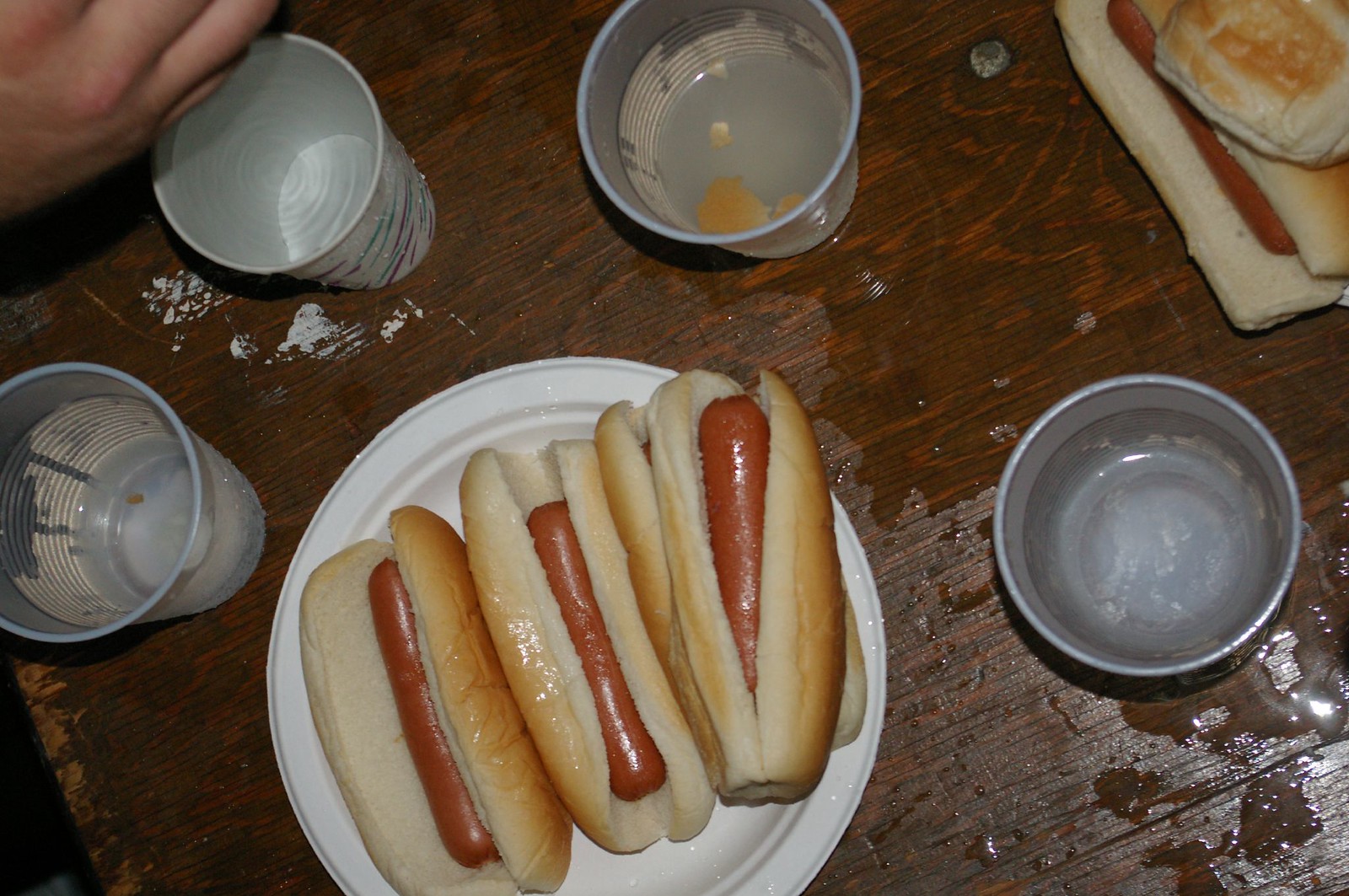A top-down view reveals a messy, dark brown wooden table with noticeable wood grain, likely in a domestic setting or a casual restaurant. Dominating the center is a white, circular thermocol plate holding four hot dogs, arranged in hot dog buns. Three hot dogs lie flat, and the fourth is stacked on top of another. Surrounding the plate, in a semi-circle, are four water-filled plastic or paper cups in varying states of fullness. Among these, one cup stands out with purple and blue stripes. Spilled liquid, possibly water, forms a substantial puddle on the right-hand side where multiple cups appear to have tipped over. In the upper right corner, there are additional hot dogs directly on the wet table, their buns soaked through. The only piece of the human element visible is a partial hand, just the back and fingers, touching the rim of a cup at the top left corner. The colors prominently seen are the brown of the buns, the red of the sausages, the silver and white of the cups, and the dark wood of the table.